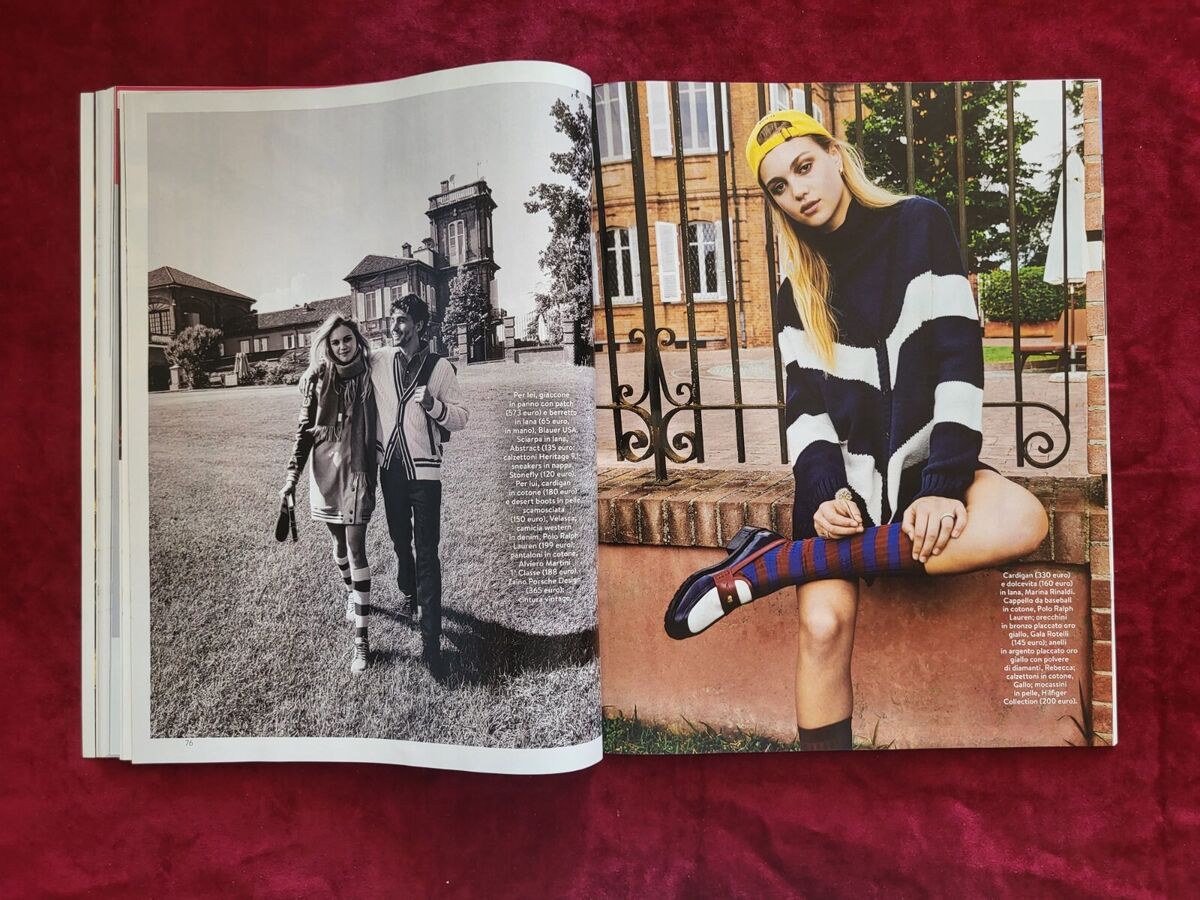The open magazine resting on a rich, red velvet cloth features a detailed spread across two pages. On the left page, the black-and-white photograph numbered 20 at the top and 76 at the bottom showcases a young man and woman walking on the lush grass in front of an elaborate two-story estate with a tower, indicative of an old college campus. The man, dressed in a white cricket sweater, black pants, and carrying a backpack over his left shoulder, has his right arm around the woman's shoulder. He is smiling and looking off to the side, while the woman, also smiling, looks directly at the camera. She is adorned in knee-high socks and holding a book, possibly also wearing a dress or coat, distinguishing her preppy and fashionable attire. 

The right page presents a vibrant color image of the same woman, now sitting cross-legged on a brick ledge with a wrought iron fence behind her. Her hair is pulled back, and she sports a yellow ball cap turned backwards. Wearing a blue sweater with two white stripes across it and likely shorts given her exposed legs, she complements her outfit with high socks bearing red and blue stripes or circles and slip-on shoes that are black with a white top and a red stripe. The ornate brick estate in the background, complete with windows, shutters, a driveway, and an umbrella or awning, provides a fittingly elaborate setting, possibly described in small, unreadable white text in the bottom left-hand corner.